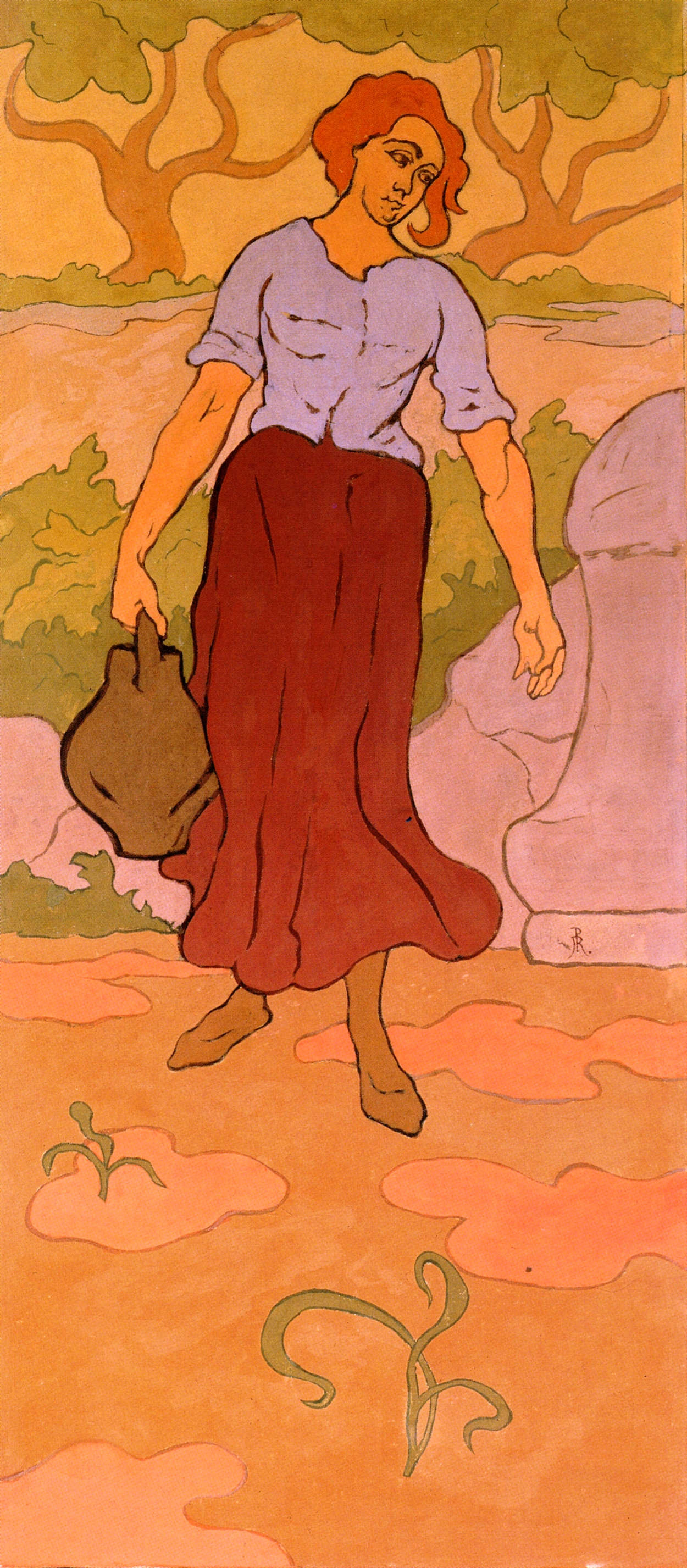This narrow vertical rectangular painting depicts a melancholic woman standing on an orangey-brown ground with two green sprouts emerging from it. The woman, with her orange/red shoulder-length hair and orangey tan skin, is dressed in a blue blouse with three-quarter-length sleeves and a long red skirt that reaches her brown boots. She appears to be carrying a brown bag, possibly a basket or water jar, in her hand, which also shows muscular arms. She is looking downwards at the ground, conveying a sense of sadness. 

Behind her, there are some gray boulders, and further back, a series of indistinct bushes and trees with brown trunks and green leafy outlines. The background transitions from the orangey ground to a sky that is a mix of orange and yellow hues. Pinkish tones are subtly present near the object she's holding. This artwork, done in a style reminiscent of colored pencil or a simple sketch, uses lines and patches of color to bring definition to the scene.